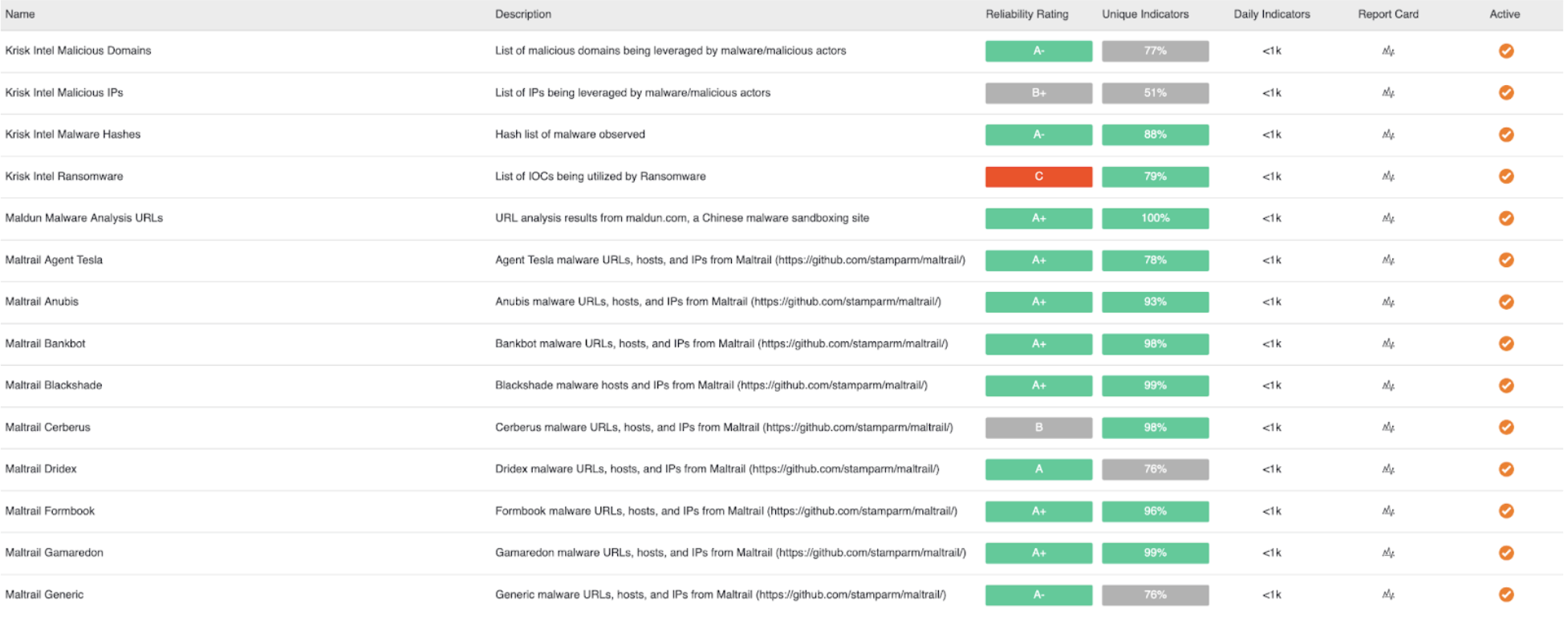This is a detailed screenshot depicting a comprehensive analysis table. Each row in the table starts with the entity's name situated on the left, accompanied by a brief description. Adjacent to the descriptions, there is a reliability rating assigned on a graded scale. The grades range from A+ to C, each highlighted with a specific background color: green for A+, gray for B, and red for C. Further to the right of the reliability ratings are unique indicators, represented as percentages ranging from 0% to 100%. These indicators are also color-coded, with values below 80% shaded in gray, while higher values are displayed in green. The table also includes columns for daily indicators and report cards, providing an at-a-glance view of performance metrics. Additionally, there is an "active" status column, which likely signifies the current operational status of each entity. The text within the screenshot is notably small, making it challenging to read the finer details without closer inspection.